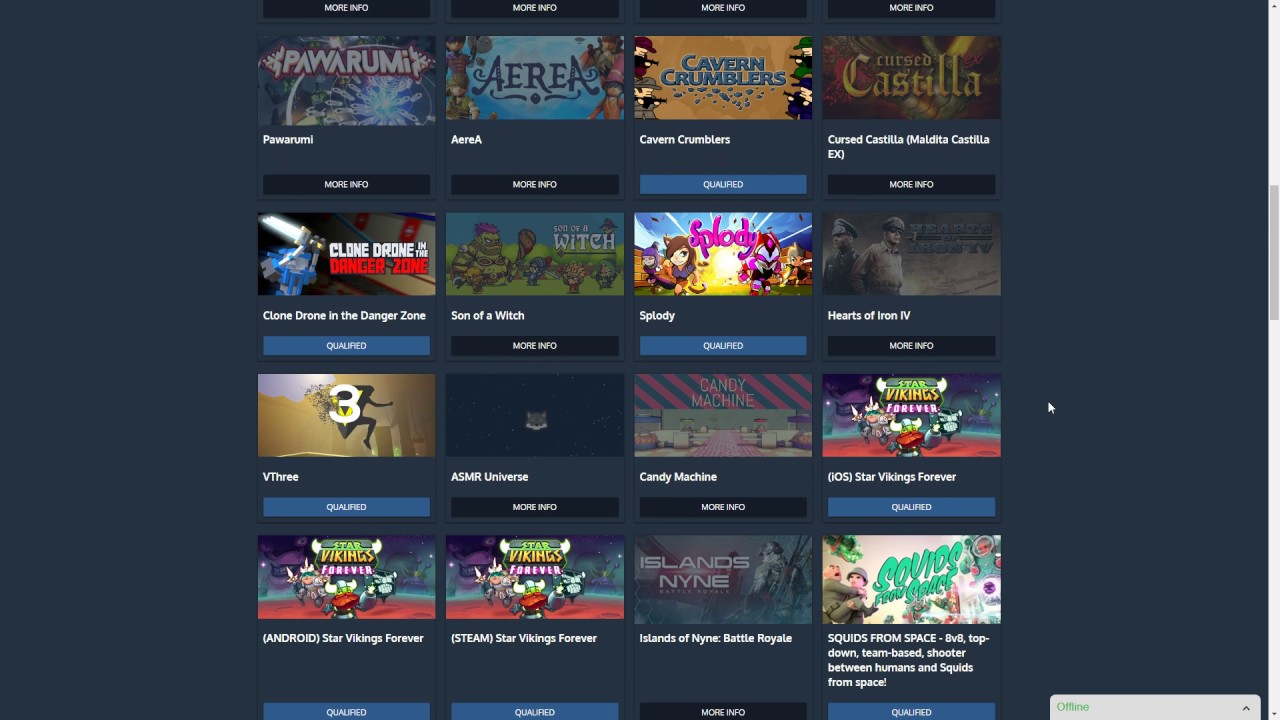The image features a dark gray, nearly black background adorned with covers of various video games organized methodically. Across the top of the page, the words "More Info" are displayed above each game title in the topmost row. This row contains four game titles arranged from left to right:

1. The first cover is rectangular and prominently displays the title "Paarumi" in large print. Below it, the word "Paarumi" appears again, confirming the game's name.
2. The second cover to the right features the title "Area." The image showcases animated characters, and beneath it, the title "Area" is repeated.
3. The third game, moving to the right, is "Cavern Crumblers," set against an orange background, depicting four characters wielding guns.
4. The fourth title is "Cursed Castilla," with the subtitle "Cursed Castilla, Maldita Castilla X" appearing below the main title.

Below this top row are pictures of four more games:

1. "Clone Drone in the Danger Zone."
2. To the right, "Son of a Witch" is displayed, featuring an image of a large ogre wielding a club alongside several other fairy tale-like characters.
3. Further right is the title "Splodey."
4. To the rightmost side is "Hearts of Iron 4," accompanied by an image of two soldiers.

Continuing to the next row of games:

1. First is "V3," showing a person running.
2. The next game is titled "ASMR Universe."
3. Following this is "Candy Machine."
4. On the far right, it says "iOS, Star Vikings Forever."

The bottom row of images contains the final four games:

1. "Android, Star Vikings Forever."
2. "Steam, Star Vikings Forever."
3. "Islands of Nine, Battle Royale."
4. Finally, "Squids from Space, an 8v8 top-down team-based shooter between humans and squids from space." 

This comprehensive layout organizes the game titles, providing visual and textual information in a structured and easily navigable format.